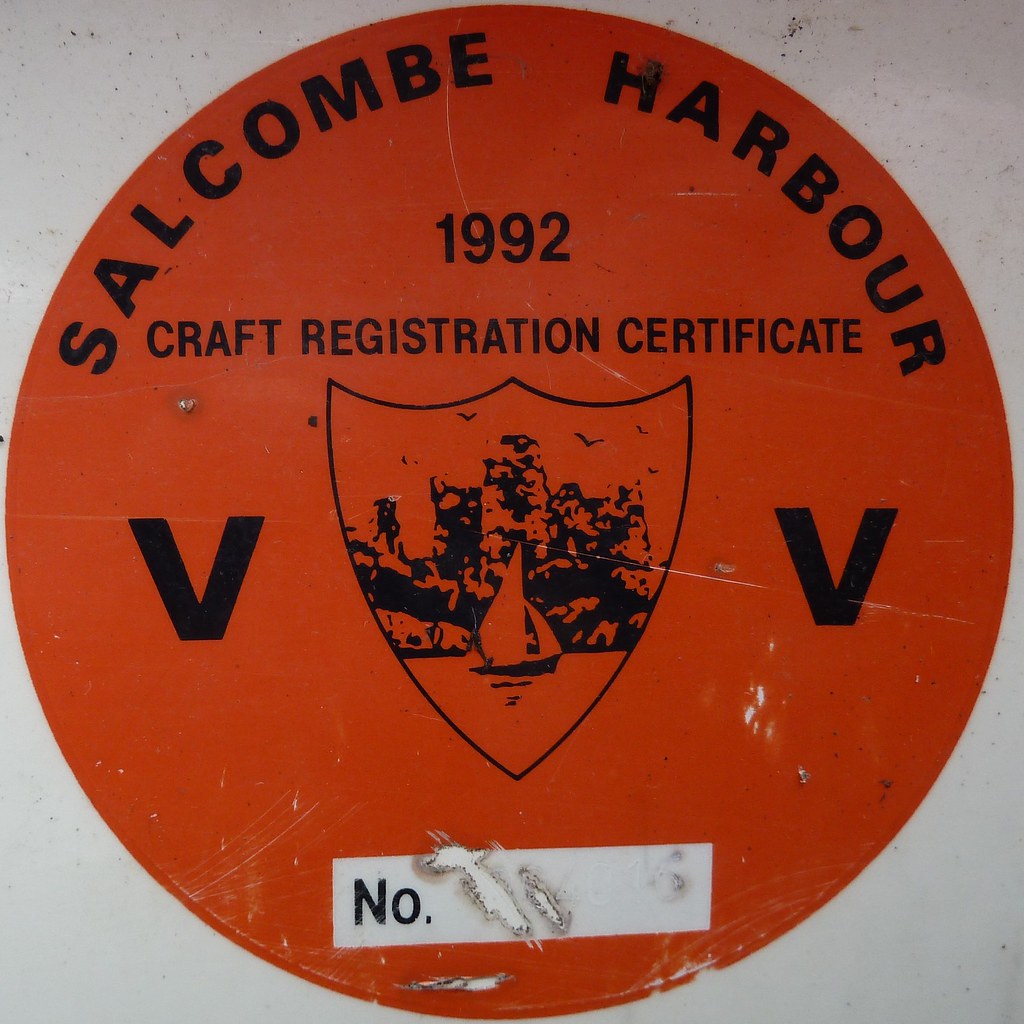This image is a color photograph in a square format with a light gray background. The photograph showcases a vintage and aged craft registration certificate from Salcombe Harbour, 1992. The certificate is circular and filled with a dark orange or red color. At the top of the circle, in black text curving along its perimeter, it reads, "Salcombe Harbour." Just below this text, and centered horizontally, are the words "1992 Craft Registration Certificate" in black print. Central to this certificate is a shield graphic depicting a sailboat on water, set against a harbor with cliffs in the background. On either side of the shield, there are bold capital letters "V" in black. At the bottom of the circle, there is a horizontal white rectangle, which contains the printing number marked as "No." in black text. This white box has visible gouges, especially on the right side, indicating wear and damage. The style of the photograph is a realistic representation of a vintage printed item, capturing its detailed textures and signs of aging.